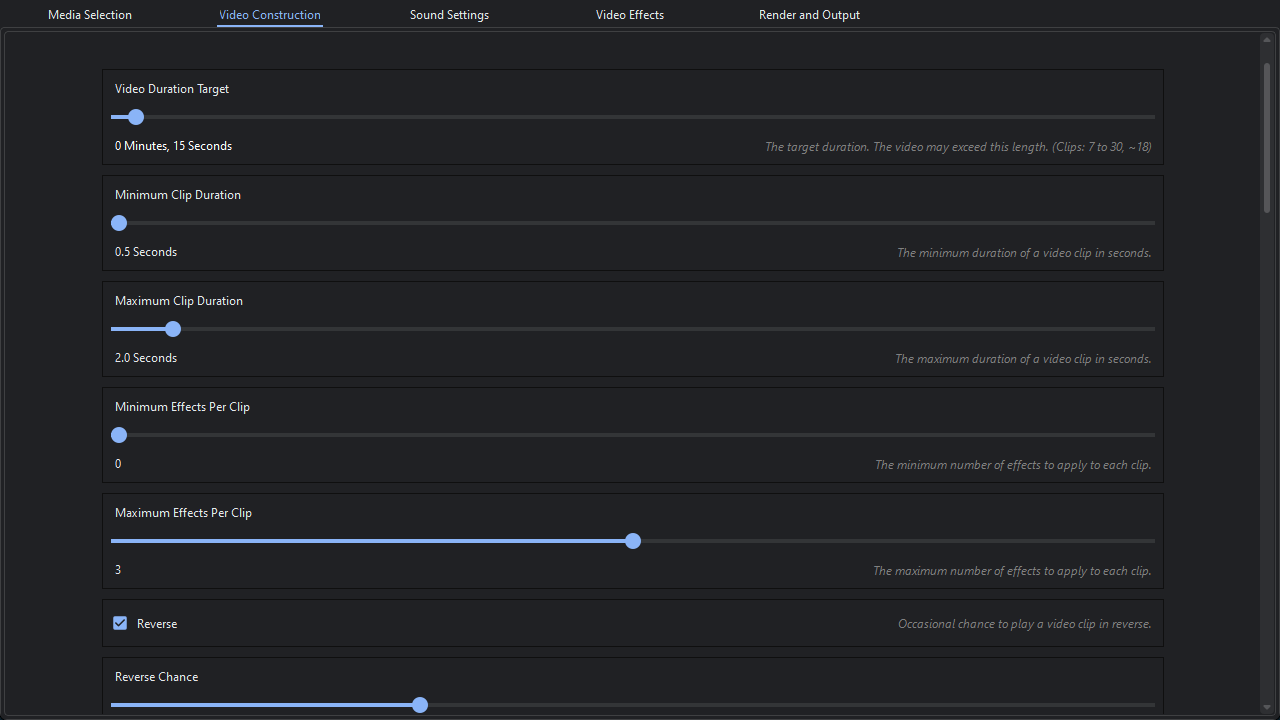Screenshot of a Video Construction Settings Page:

The image showcases a screenshot of a settings page with a sleek black background and white text. The top section features a selection of different settings categories, including 'Media Selection', 'Video Construction', 'Sound Settings', 'Video Effects', 'Render', and 'Output'. The 'Video Construction' tab is currently selected, highlighted by blue text and an underline.

The settings displayed on this page are as follows:

1. **Video Duration Target**:
   - Set to: 0 minutes and 15 seconds
   - Description: "The target duration. The video may exceed this length, clips 7 to 30, about 18."

2. **Minimum Clip Duration**:
   - Set to: 0.5 seconds
   - Description: "The minimum duration of a video clip in seconds."

3. **Maximum Clip Duration**:
   - Set to: 2.0 seconds
   - Description: "The maximum duration of a video clip in seconds."

4. **Minimum Effects per Clip**:
   - Set to: 0
   - Description: "The minimum number of effects to apply to each clip."

5. **Maximum Effects per Clip**:
   - Set to: 3
   - Description: "The maximum number of effects to apply to each clip."

6. **Reverse**:
   - Selected (box is checked)
   - Description: "Occasional chance to play a video clip in reverse."

7. **Reverse Chance**:
   - Partially clipped out from the image, making it unreadable.

In the middle of the settings options, certain elements, such as option bars, are highlighted in blue for better visibility.